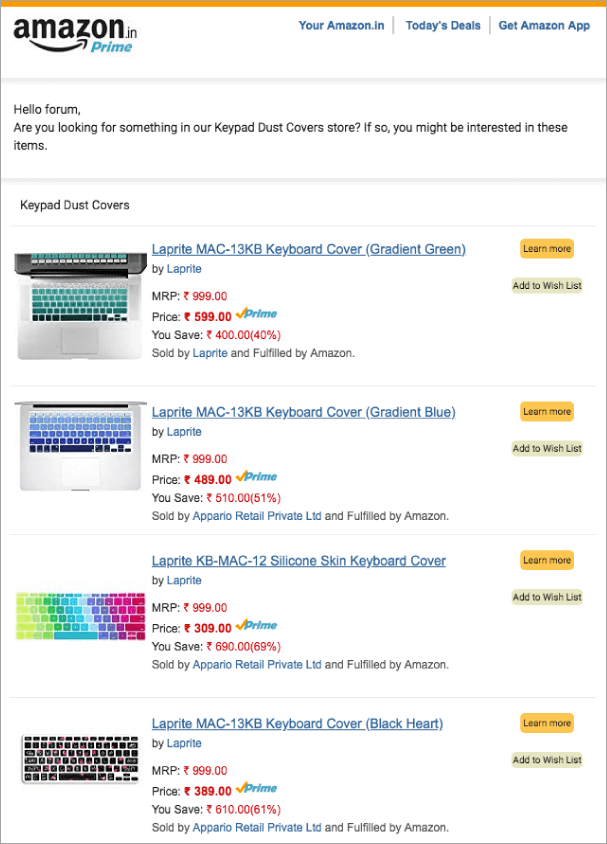**Caption:**

This image depicts a webpage from the Amazon India site featuring a selection of suggested products. In the top left corner, the page displays a greeting and inquiry: "Hello, Forum. Are you looking for something in our Keypad Dust Cover store?" It then directs users to a curated list of items under the category "Keypad Dust Covers." 

The main content showcases four products, each accompanied by a detailed description. Here, from the top down, are the items shown:
1. **LapRite Mac 13KB Keyboard Cover, Gradient Green** - shown with an image of the product, displaying its seller, suggested price, Amazon's price, savings, and fulfillment details.
2. **LapRite Mac 13KB Keyboard Cover, Gradient Blue** - identical to the first product but with a different gradient color.
3. **LapRite KB Mac 12 Silicone Skin Keyboard Cover, Rainbow** - featuring a vibrant, multi-colored design and sold by LapRite.
4. **LapRite Mac 13KB Keyboard Cover, Black Heart** - a sleek, black cover sold by Aperio Retail Private Limited and fulfilled by Amazon.

Each product listing includes interactive buttons for "Learn More" and "Add to Wish List," enabling an engaging and detailed shopping experience.